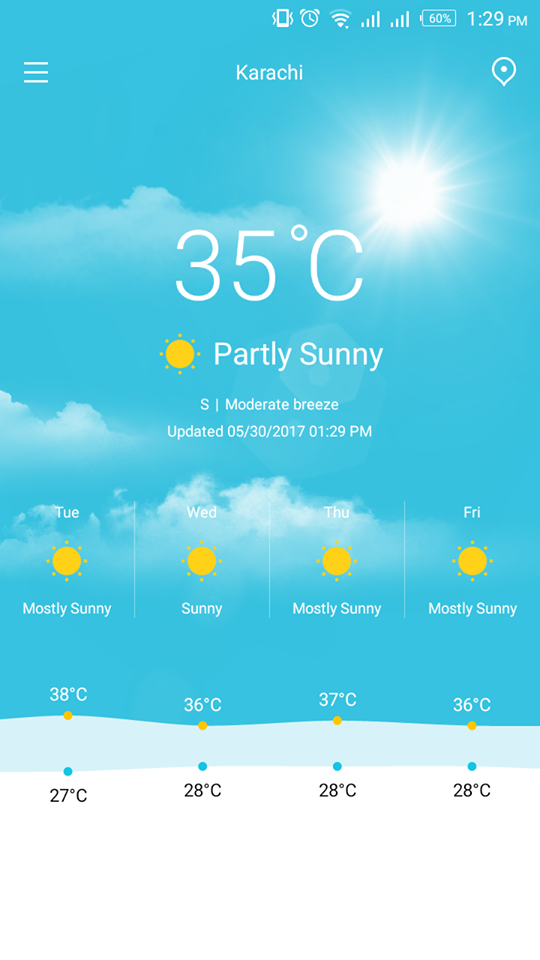Screenshot of a smartphone display shows the current weather and various phone status icons in Karachi, August 5, 2017, at 1:29 PM. The status bar at the top right corner indicates the phone is on vibrate mode, the alarm is set, Wi-Fi is connected, and the network signal is present, with the battery at 60%. Below the status bar, "Karachi" is displayed against a backdrop of a bright blue sky with scattered clouds and a shining sun.

The current weather reading shows 35°C and partly sunny, with a moderate breeze. The specific weather update was last refreshed at 1:29 PM on Tuesday. The forecast for the upcoming days includes:
- Wednesday: Sunny, high of 36°C, low of 28°C.
- Thursday: Mostly sunny, high of 37°C, low of 28°C.
- Friday: Mostly sunny, high of 36°C, low of 28°C.

This vertical image lacks any human presence, animals, plants, vehicles, or buildings, emphasizing the digital display and weather information.